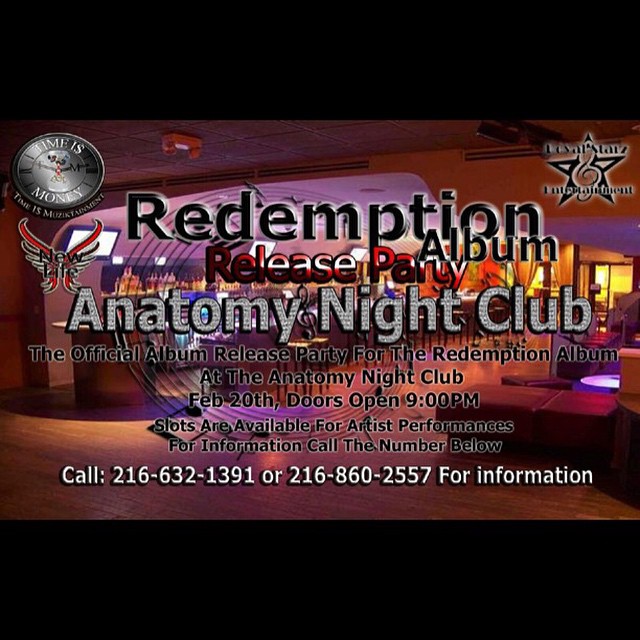The image features a vivid promotional banner for the "Redemption Album Release Party" at Anatomy Nightclub, set against a dimly lit backdrop that hints at an outdoor bar or club entrance adorned with purple, red, orange, and yellow hues. The central text, prominently displayed an inch and a half from the top, announces the event details: "Redemption Album Release Party, Anatomy Nightclub," emphasizing its significance as the official release celebration for the Redemption album. Scheduled for February 20th, doors open at 9 p.m. The banner invites artists to book performance slots and provides two phone numbers for contact. In the upper left corner, there's a symbol encircled by the phrase "Time is Money," possibly indicative of "Time is Money Entertainment," and in the upper right corner, a logo featuring a star and ampersand, likely for "Royal Stars Entertainment." The overall scene blends the festive atmosphere with detailed event information to entice party-goers and performers alike.